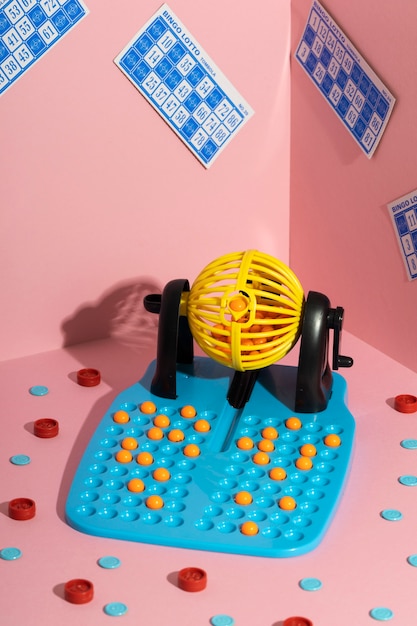This photograph captures the intricacies of a bingo lotto game setup. Central to the image is a detailed shot of the mechanical bingo machine, made of plastic. A large yellow spherical cage at the machine's core holds numerous smaller balls used for the game. Attached to this central cage is a black crank, which, when rotated, releases one ball at a time. These balls descend into individual slots on a blue plastic tray connected to the crank. The setup rests on a pink surface, adorned with scattered red and blue circular bingo chips. The background features right-angled pink walls, embellished with four bingo lotto cards, illustrating the game's playing format. This vibrant scene vividly showcases the engaging elements of a classic bingo game in progress.